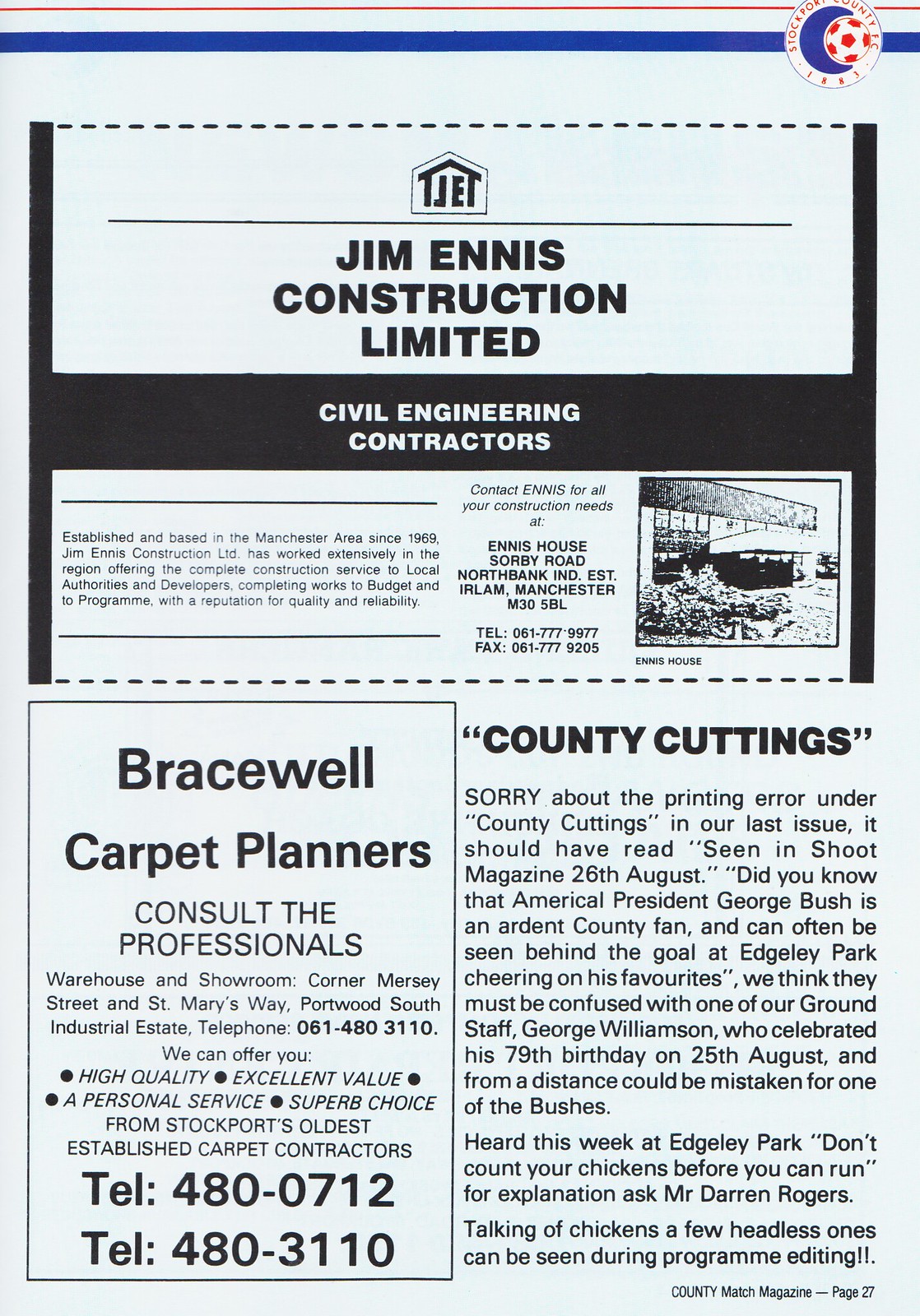The image is a page from a magazine with a light blue-tinted background. At the top, a thin orange bar is followed by a slightly larger blue bar. The upper right side features a white-outlined circle with red text that partially reads "Stockton," enclosing another blue circle with a soccer ball that has orange and white spots, offset to the left. Beneath this, a black dotted line extends horizontally across the page, intersected by vertical black lines, and below it, there is a solid black line.

Centered at the top of the page, bold text on a white background reads "Jim Ennis Construction Limited." Directly below, a black bar with white text states "Civil Engineering Contractors." Further down, a paragraph details the company's extensive work in the Manchester area since 1969, emphasizing its reputation for quality and reliability. Directly to the right, contact information for Jim Ennis Construction Limited is provided, listing the address as Ennis House, Sorby Road, North Bank, IND. EST, Irlam, Manchester, M305BL, and telephone and fax numbers (061-777-9977 and 061-777-9250).

On the right side of the section, there's an outline of an old building with the caption "Ennis House" below it. Further down the page, an old black and white photograph shows a building being demolished.

The bottom left corner features an advertisement for Bracewell Carpet Planners, emphasizing their professional consultancy, warehouse, and showroom located at the corner of Mersey Street and St Mary's Way, Portwood South Industrial Estate, with phone numbers 480-0712 and 480-3110. Adjacent to this, a rectangular bordered column promotes their high-quality service and significant choice.

In the bottom right corner, the page includes a segment titled "County Cuttings" in bold. The text humorously addresses a printing error from a previous issue and relates an amusing anecdote involving American President George Bush and a lookalike at Ackley Park. It concludes with a reference to some headless chickens seen during program editing, adding a light-hearted touch. At the very bottom, the page is marked as part of the "County Match Magazine" on page 27.